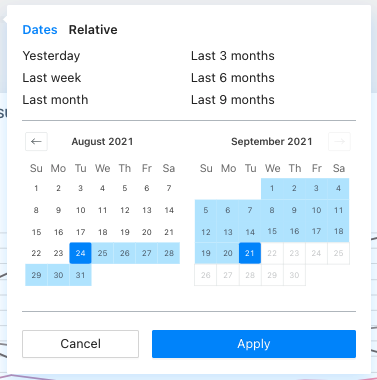The image is a screenshot of a website interface that allows users to select different date ranges. At the top left corner in blue text, it reads "Dates." The options available include "Relative," with subsequent selections listing "Yesterday," "Last Week," "Last Month," "Last Three Months," "Last Six Months," and "Last Nine Months." Below these options, there are two calendar displays for selecting specific dates: one for August 2021 and the other for September 2021. At the bottom of the interface, on the left side, there is a gray "Clear" or "Cancel" button, and on the bottom right side, there is a blue "Apply" button.